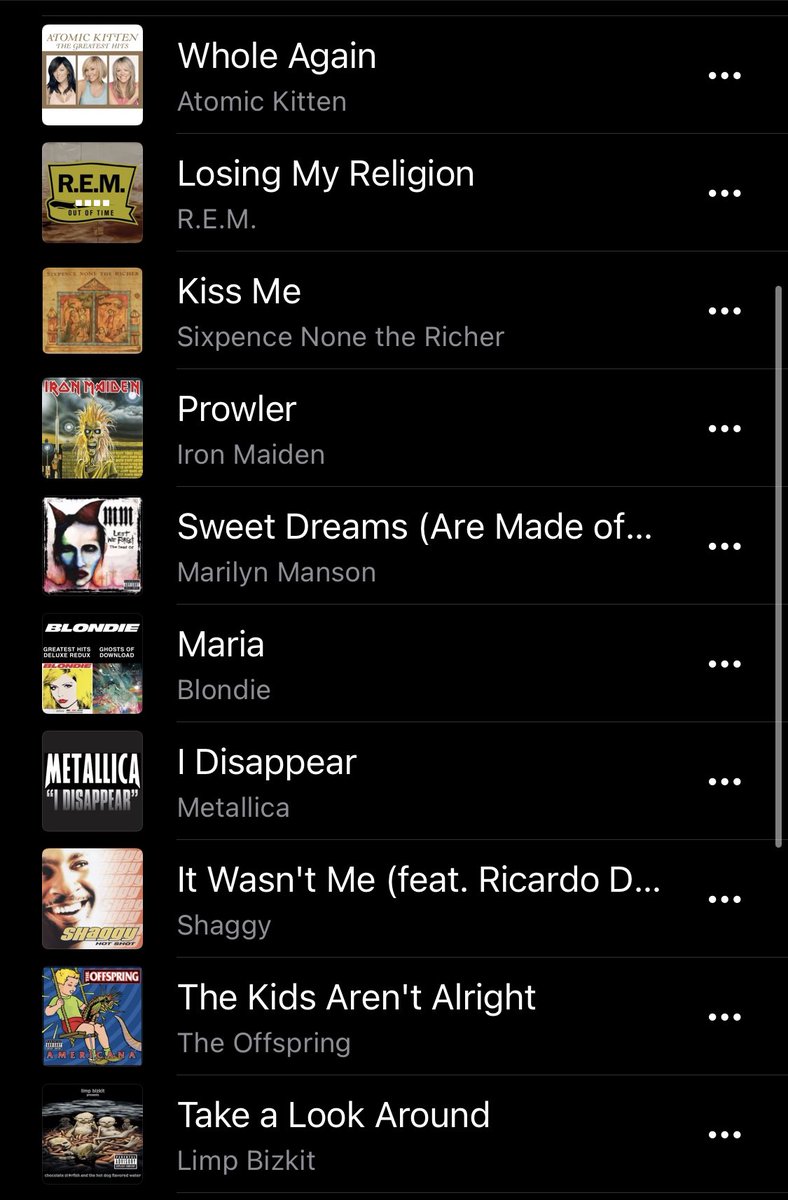This is a detailed screenshot of a mobile device, either a phone or tablet, displaying a music library interface in portrait mode with a black background. On the right side of the screen, there is a vertical, gray, rounded scroll bar situated centrally. Additionally, there are multiple vertically aligned three-dot option buttons running the full length of the image, also on the right-hand side.

On the left side of the screen, colored album covers are aligned vertically, with corresponding titles of songs and artists occupying the center section of the display, creating orderly rows. The text descriptions are white for song titles and gray for artist names set against the black background.

From top to bottom, the listed songs and artists are as follows:
1. "Hole Again" by Atomic Kitten
2. "Losing My Religion" by R.E.M.
3. "Kiss Me" by Sixpence None the Richer
4. "Prowler" by Iron Maiden
5. "Sweet Dreams (Are Made of This)" (cut off) by Marilyn Manson
6. "Maria" by Blondie
7. "I Disappear" by Metallica
8. "It Wasn't Me" featuring Diddy D (cut off) by Shaggy
9. "The Kids Aren't Alright" by The Offspring
10. "Take a Look Around" by Limp Bizkit

The album covers on the left are vividly colored, providing a striking visual contrast to the monochromatic text descriptions in the center. The interface design is straightforward, focusing on a simple layout that clearly displays song and artist information.